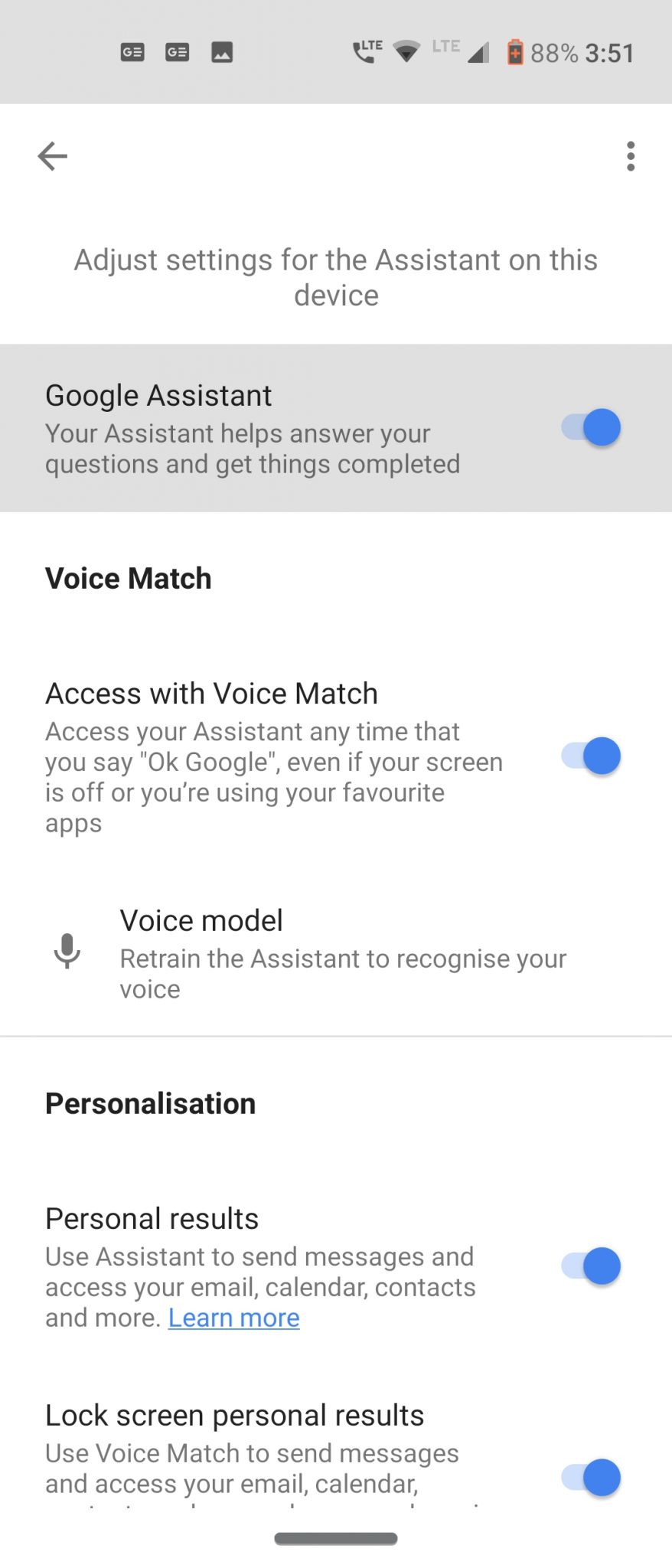A mobile phone screen displays a web page, with the current time shown as 3:51 PM at the top. The battery life indicator reads 88%, and the signal strength shows full bars. A voicemail notification is also visible. The interface features a minimalist design with gray and black text on a white background. 

At the very top of the screen, a back arrow icon is situated on the left, while three vertical dots for more options are located on the right. Below this, a gray ribbon with black text reads "Google Assistant." Just beneath, in gray text, is the description: "Your assistant helps answer your questions and get things completed."

An option to adjust the assistant's settings is turned on, indicated by a blue toggle switch. Following this, the "Voice Match" feature is described in black text on a white background: "Access with Voice Match. Access your assistant any time that you say 'OK Google,' even if your screen is off or you're using your favorite apps." This feature is also enabled, as shown by another blue toggle switch.

Further down, a section titled "Voice Model" in black text with a microphone icon instructs users in gray text: "Retrain the assistant to recognize your voice."